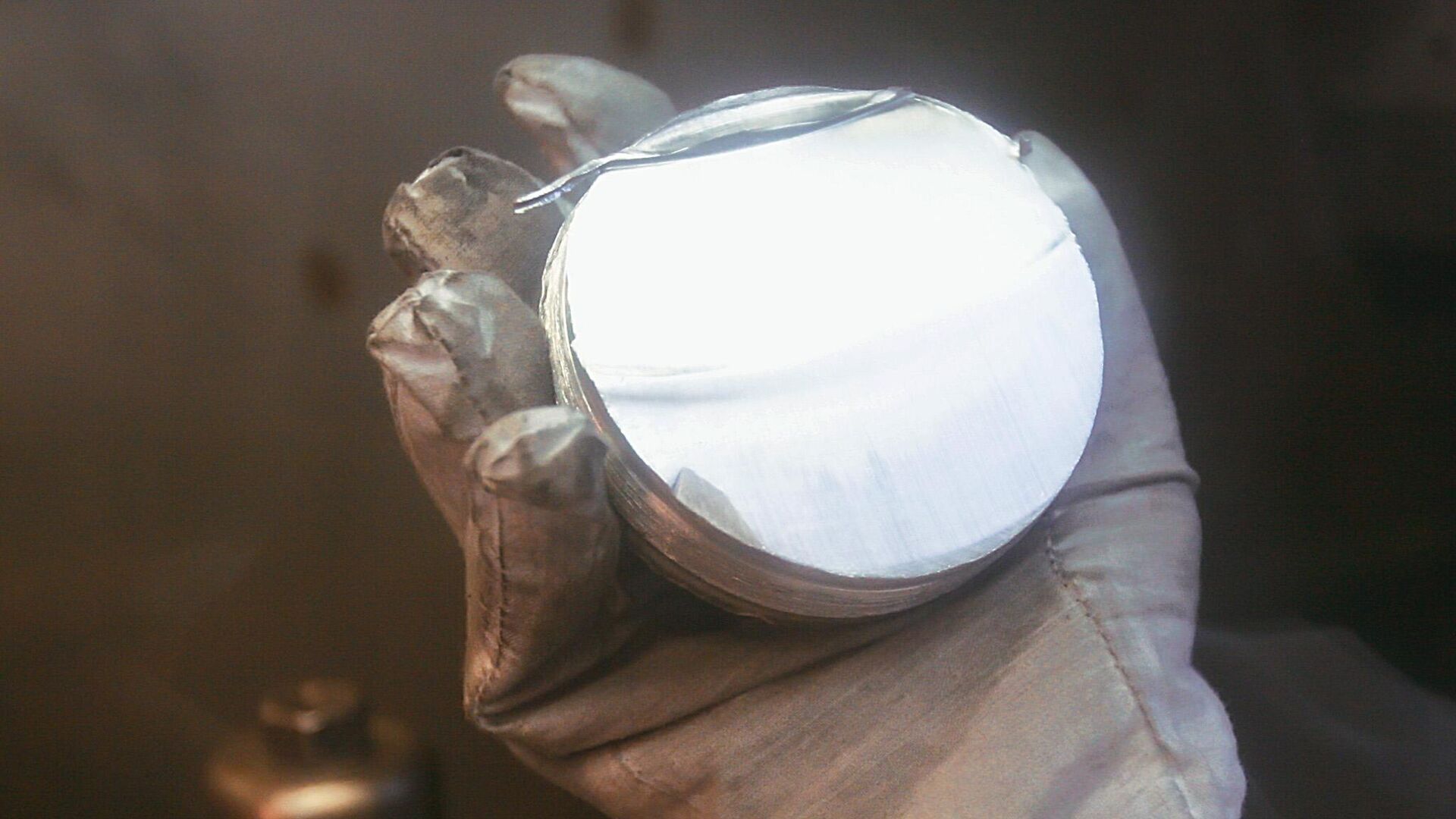The photograph features a landscape-oriented shot, approximately 1.5 times wider than it is tall. At the center of the image is a right hand, palm facing up, adorned with a thick, heavily-stitched glove that appears silvery gray. This glove is likely designed for handling high-heat or hazardous materials, as indicated by its reinforced, protective nature. The gloved hand is holding a circular metallic object that resembles a bisected sphere; the exposed flat side mirrors its surroundings, suggesting a shiny, almost tinfoil-like surface. Some foil appears to be loose, hinting that it might be peeled away later. The background is unfocused and predominantly dark, blending from brown on the left to black on the right. Additionally, on the bottom left, there is a blurry, open canister, though its contents are indiscernible due to the lack of focus.